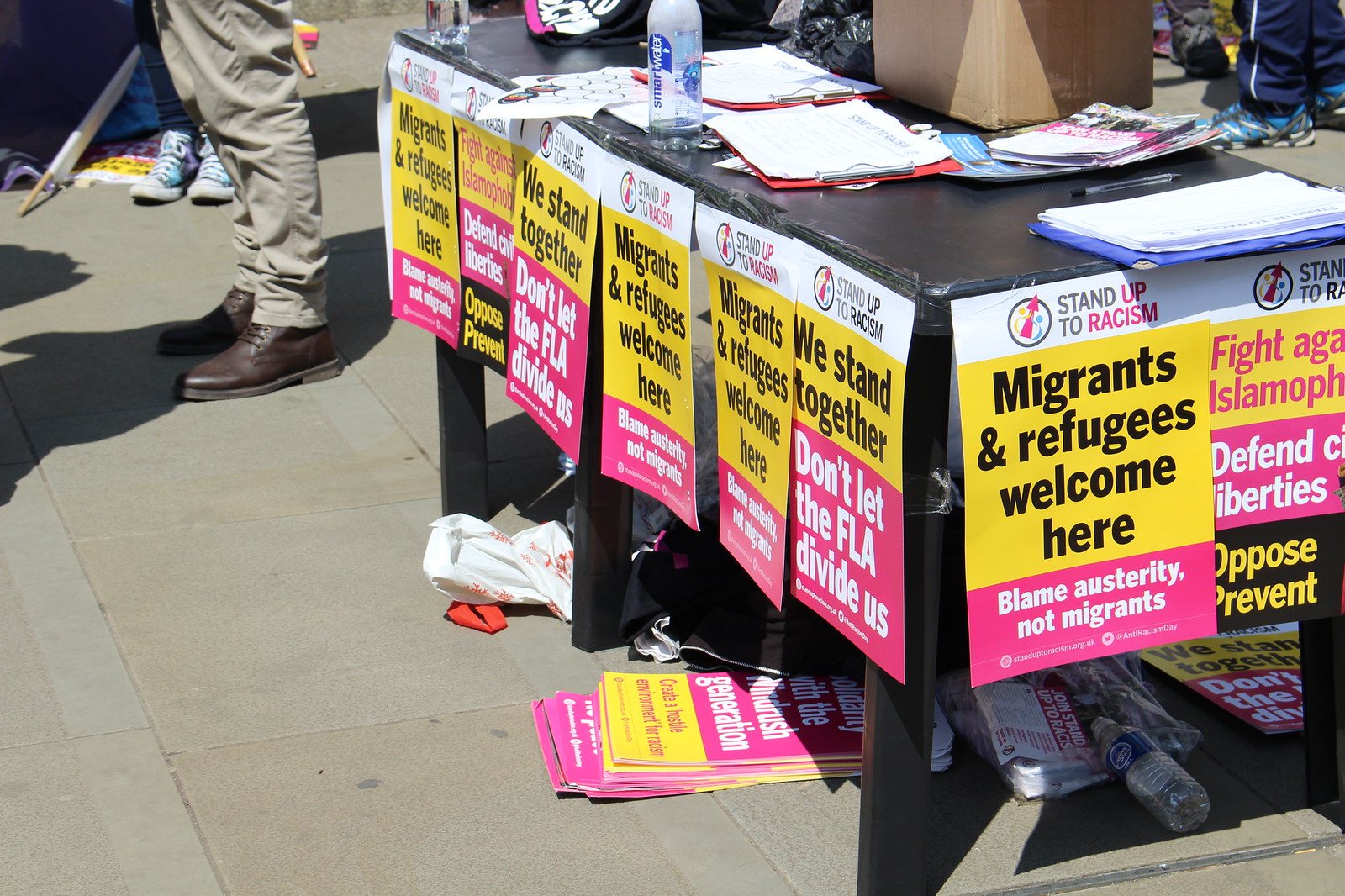The image depicts an outdoor setup on a concrete surface, with bright sunlight and shadows suggesting it was taken during the daytime. Central to the scene is a black table with three legs on each end, laden with various items including pamphlets and flyers, all aligning with an anti-racism theme. The materials prominently display messages such as "Stand up to racism," "Migrants and refugees welcome here" in bold black font on a yellow background, "Blame austerity not migrants" in white text on pink, and "We stand together, don't let the FLA divide us." 

There are multiple sets of these posters, some of which are taped around the table and others stacked beneath it. The table itself holds a cardboard box, a large Smart water bottle, various papers, and several clipboards in red and blue. Nearby, you can see the lower halves of people standing, one wearing blue shoes with white soles and another in light beige pants with brown shoes, holding something behind their legs. The setting feels like a concrete sidewalk or parking area, adding to the community-organized vibe of the scene.